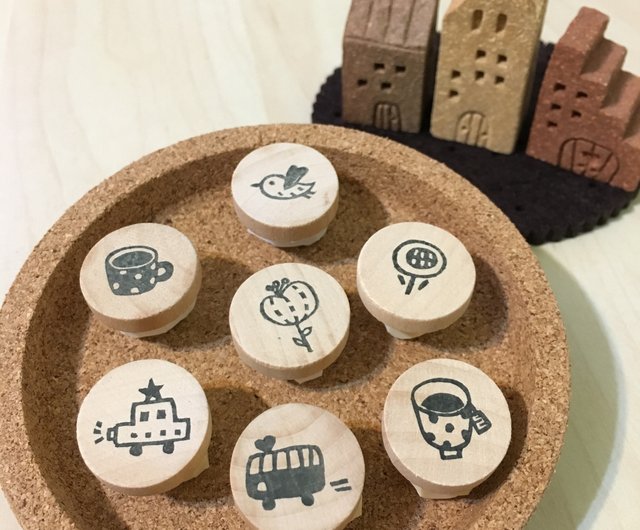The image depicts a child's puzzle or toy that resembles a coaster in shape. The main feature is a wooden base with indentations designed to hold small, round, carved wooden buttons. Each button has a picture on it, facing upward, with some space surrounding them. In the center, there is one button with sticks radiating outward. 

The illustrations on the buttons include:
- A bird positioned at the top.
- A round flower located to the right, following a clockwise direction.
- A coffee cup placed underneath the flower.
- A bus at the bottom featuring a heart symbol.
- An ambulance situated to the left of the bus.
- Another cup, possibly filled with hot chocolate and adorned with dots, above the ambulance.

The object resembles a shallow bowl or coaster made of cork, appearing short and flat on the top with some empty space. In the upper right-hand corner, there are carvings that appear to be small buildings, possibly made of clay or resembling bricks, with holes representing windows and carved doors. 

Both the cork object and the small buildings rest on a light-colored wooden table. The image is cut off at the bottom, the top, and partially on the left side.